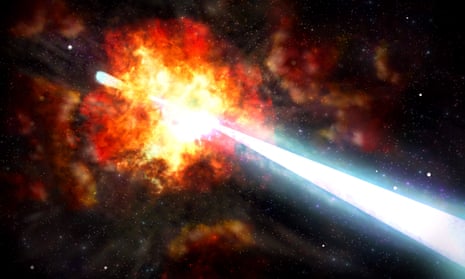The image depicts a dramatic scene in deep space, potentially a computer-generated blend with a photograph, showcasing a vivid astronomical event. The primary background is a deep black, studded with numerous stars, evoking the vastness of outer space. The focal point, slightly off-center to the left, is a colossal, fiery explosion that radiates outward in concentric layers of color: a white-hot core that diffuses into yellow, red, and fiery orange hues. Piercing through the middle of this explosion is a brilliant white beam of light, originating from the bottom right corner and narrowing as it intersects the explosion’s core, resembling a lightsaber slicing through the chaos. This beam refracts various colors, including shades of red, orange, yellow, green, indigo, and violet, adding to the surreal and vibrant spectacle. Emerging from this point of collision are several clouds and spurts of gas, blending into the cosmic backdrop. To the right of the explosion, at a similar angle to the beam, a comet streaks away with a white body and a light blue tip, trailing remnants of the explosive aftermath. This intricate tableau captures the intensity and beauty of a cosmic event, likely involving the collision of astral objects.